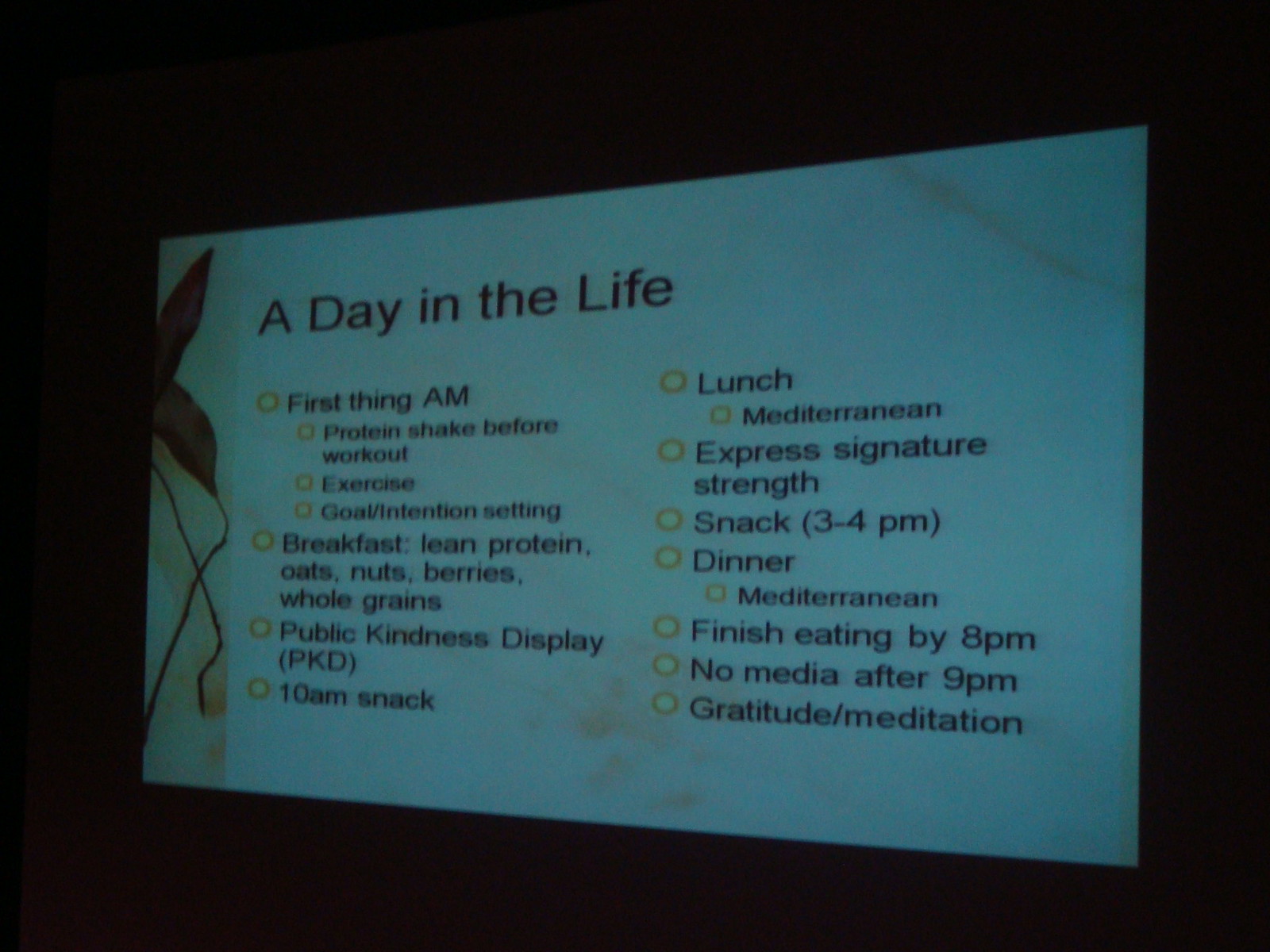The image depicts a slightly angled photo of a PowerPoint presentation slide, taken from a position off to the right. The presentation screen has a marbled white background and is bordered in black, with the rest of the surrounding area being dark. On the left side of the slide, there is a decorative plant. The slide header, titled "A Day in the Life," is followed by various activities and dietary details listed with yellow bullet points and black text. The detailed list includes: starting the day with a "protein shake before workout," followed by "exercise" and "goal intention setting." Breakfast consists of "lean protein, oats, nuts, berries, and whole grains." There is a "public kindness display (PKD)" shortly after. A "10 a.m. snack" precedes lunch, which is described as "Mediterranean." The afternoon continues with expressing "signature strength" and a snack between "3 to 4 p.m." Dinner is again described as "Mediterranean," with the note to "finish eating by 8 p.m." The day concludes with "no media after 9 p.m." and "gratitude/meditation."